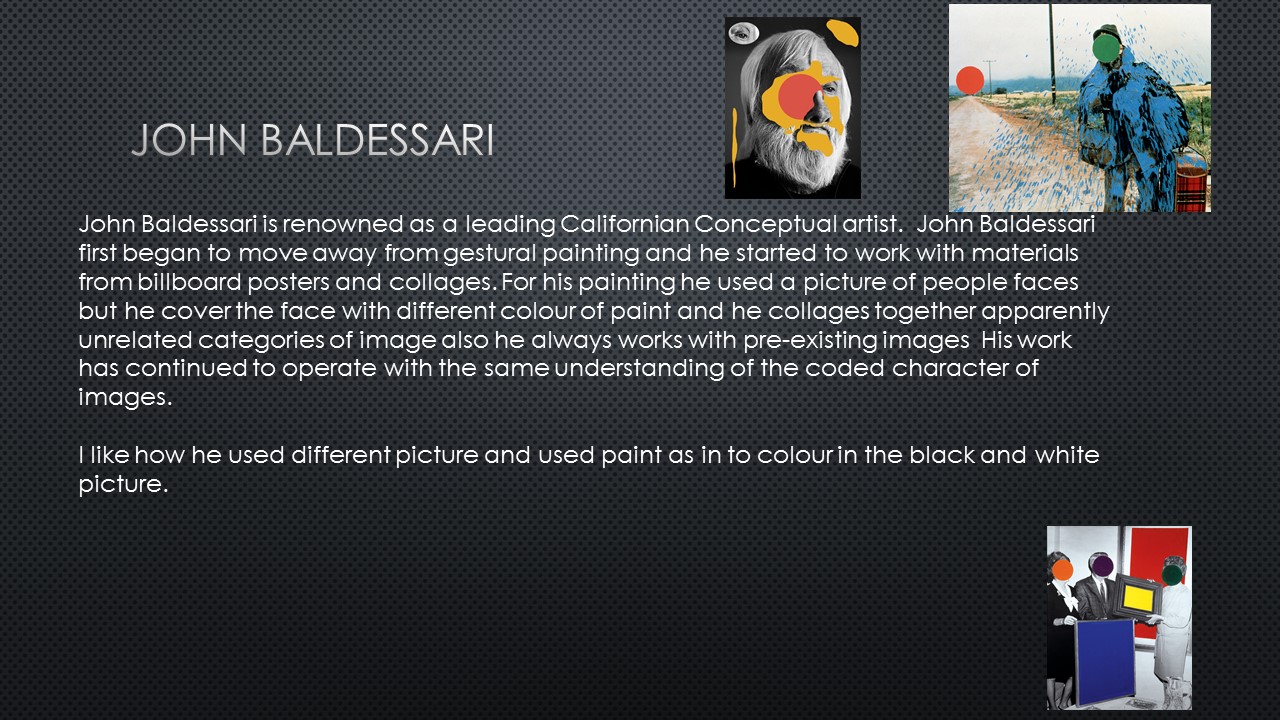The image is a depiction of a webpage or possibly a slide from a slideshow, featuring a black and gray pixelated background. Prominently displayed in white lettering at the top left are the words "John Baldessari," followed by a brief description: "John Baldessari is renowned as a leading Californian conceptual artist." The text continues beneath, detailing Baldessari's artistic evolution, noting that he transitioned from gestural painting to incorporating materials from billboard posters and collages. He frequently used pre-existing images of people's faces, which he obscured with colorful paint, creating a stark contrast against the black and white backdrop. This technique, combining unrelated categories of images, underscores his exploration of the coded character of images. The right side of the image showcases three of Baldessari's artworks, characterized by vibrant blotches of color covering the faces in the photographs. These artistic pieces are an example of his unique style, where he layered colorful shapes over black and white images, enhancing the visual narrative and conceptual depth of his work.